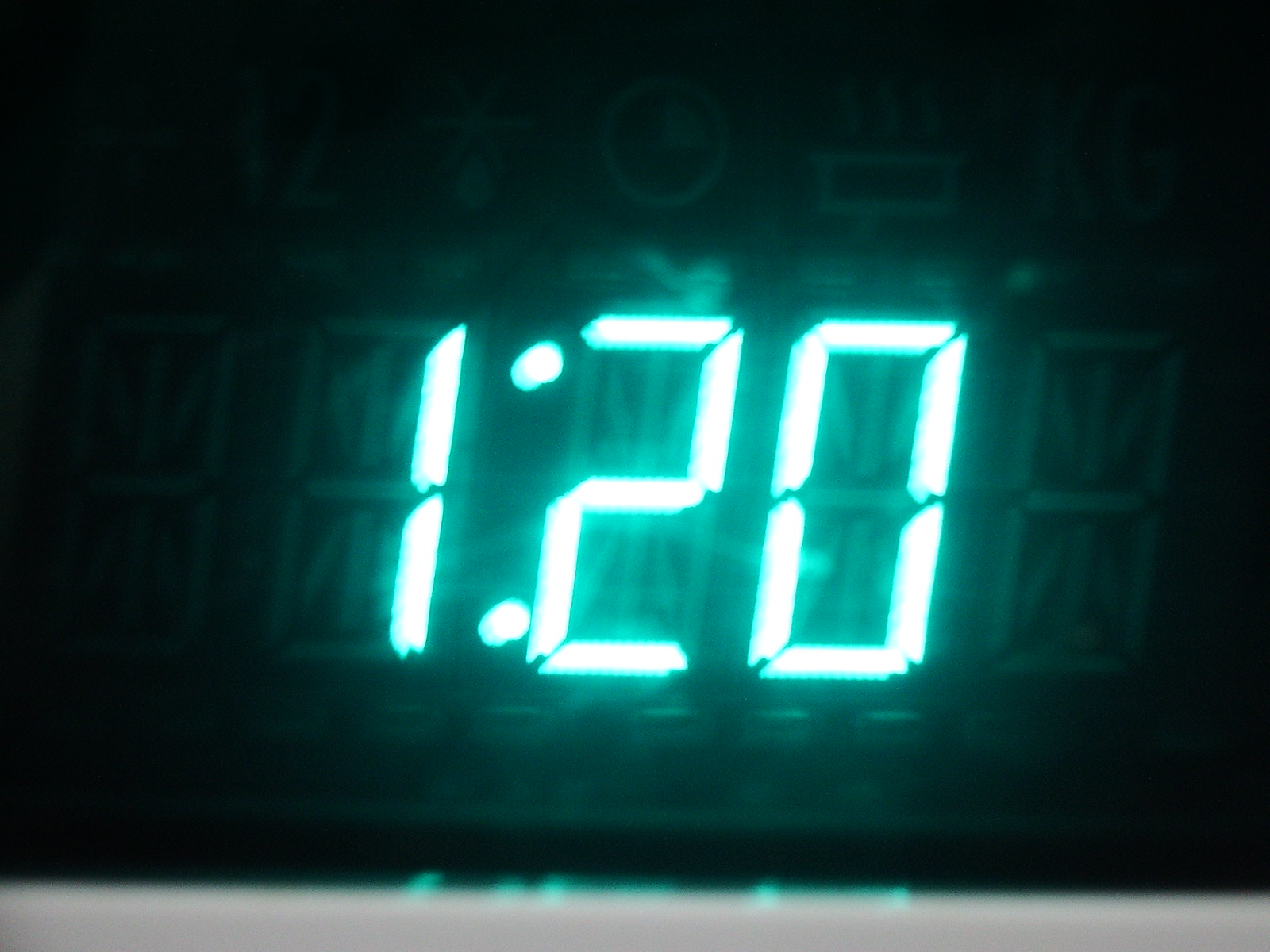The photograph captures an extreme close-up view of a digital clock displaying the time 1:20. The illuminated numbers appear predominantly white with a faint green-blue hue around their edges. The clock itself isn’t visible, leaving only the glowing digits against a dark backdrop. This close perspective allows us to see the ghostly outlines of potential numbers that could be displayed when different segments light up. The background remains mostly black, with some faint, blurry icons and a greyish strip along the bottom, adding minimal context to the image. The overall effect is slightly blurred, emphasizing the ethereal glow of the digital display.